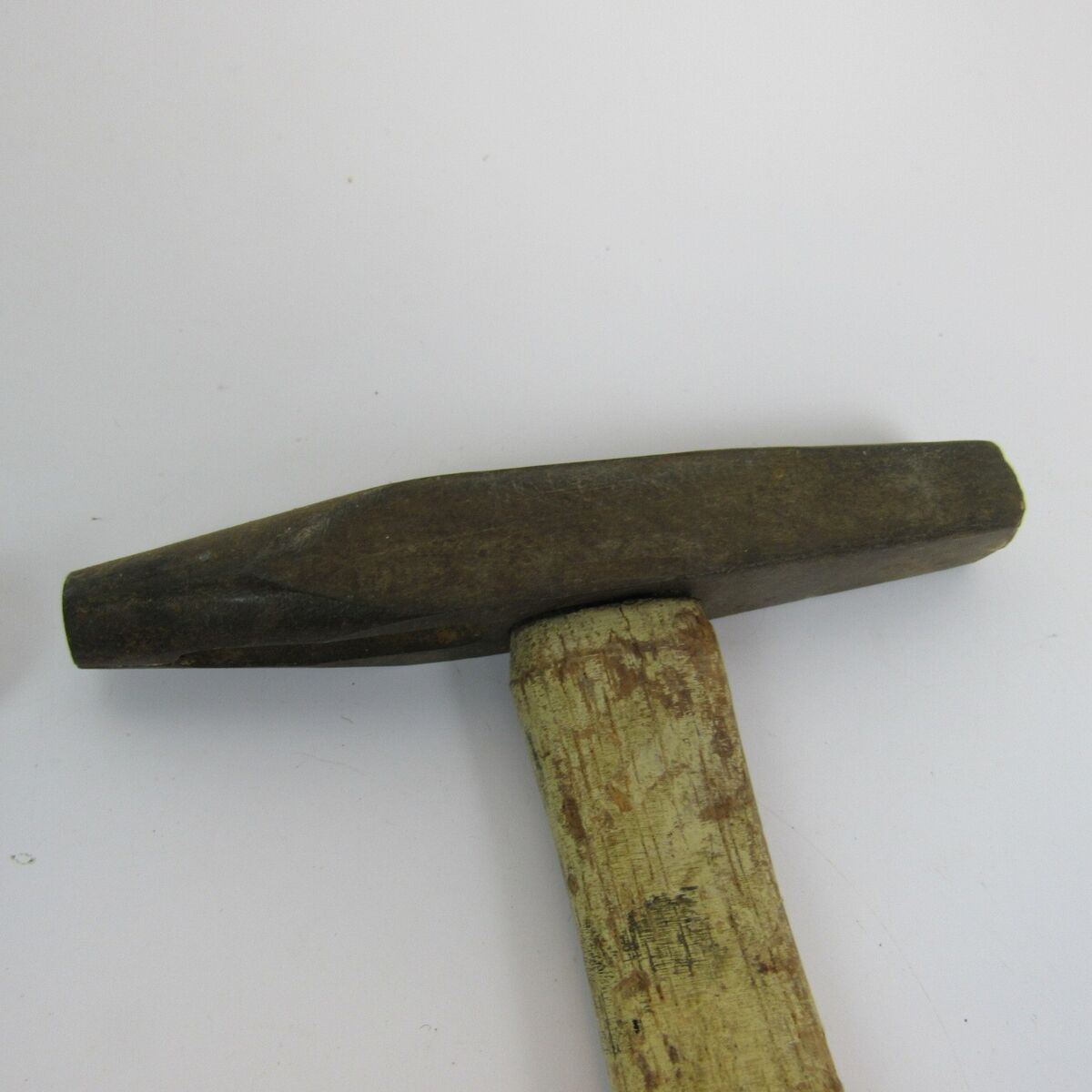This close-up, square photograph features an extremely weathered, 19th-century railroad hammer against a white background. The hammer's wooden handle, extending about six inches downward from the head and showing signs of old, flaking yellow paint, is partially visible. Black smudges and the exposed wood underneath add to its antique appearance. The hammer’s metal head is a long, narrow rectangle of steel, worn and age-tarnished with a slight brown tinge. One side of the head is flat, presumably for striking, while the other tapers into a subtly circular, quasi-pointed end, though it is not sharp. Both ends of the metal head show significant wear, emphasizing its age and extensive use.